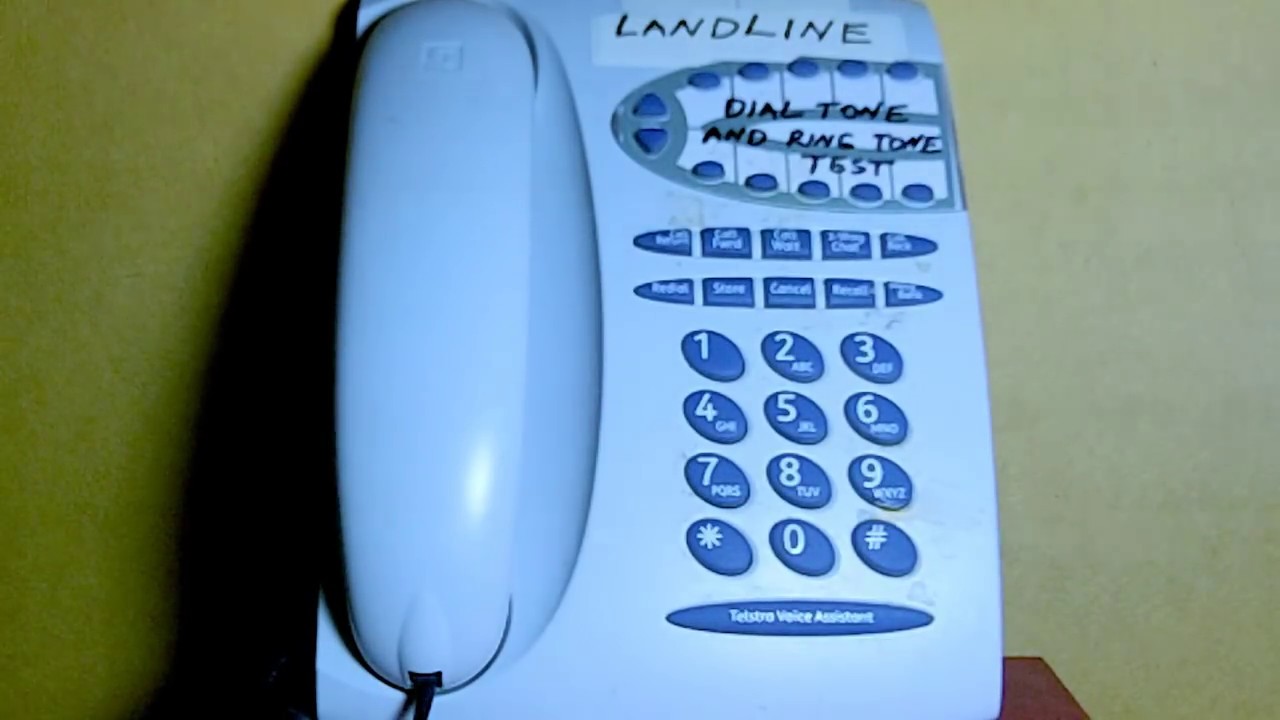This image features an old-fashioned touch-tone landline telephone, prominently centered against a mustard brown background that transitions from a darker shade on the left to a lighter shade on the right. The phone itself is white with blue pushbuttons, and it occupies the entire upper and lower sections of the photo, casting a subtle shadow on the left side of the backdrop. 

The design of the phone is reminiscent of the 90s, with a rounded brick-style receiver resting in an indented cradle. A black cable connects the handset to the receiver base. At the top right of the phone's main body, there's a white sticker with "LANDLINE" hand-written in black, capital letters. Below the sticker, there is an arc-shaped arrangement of buttons marked for volume control and speed dial functionalities. The arc is adorned with five blue buttons.

Underneath the arc, text in black, all caps reads "DIAL TONE" and "RING TONE TEST." Following this text, there are two rows of oval-shaped buttons designated for speed dialing. The buttons are blue with white block letter labels. Further down, there are additional lines of blue buttons that form an oval shape horizontally, each labeled with white text indicating numbers and corresponding letters for dialing: 

- The first row includes numbers 1, 2 (with letters A, B, C), and 3 (D, E, F)
- The second row includes numbers 4 (G, H, I), 5 (J, K, L), and 6 (M, N, O)
- The third row includes numbers 7 (P, Q, R, S), 8 (T, U, V), and 9 (W, X, Y, Z)
- The final row consists of symbols: asterisk (*), zero (0), and pound (#)

Beneath these numeric buttons lies a long oval button labeled "TELSTRO VOICE ASSISTANT" in white against the blue background. The telephone is situated on a brown table, suggesting the setting is likely inside a house. Overall, the photo captures a nostalgic piece of technology with detailed labeling and distinct colors, characteristic of its era.